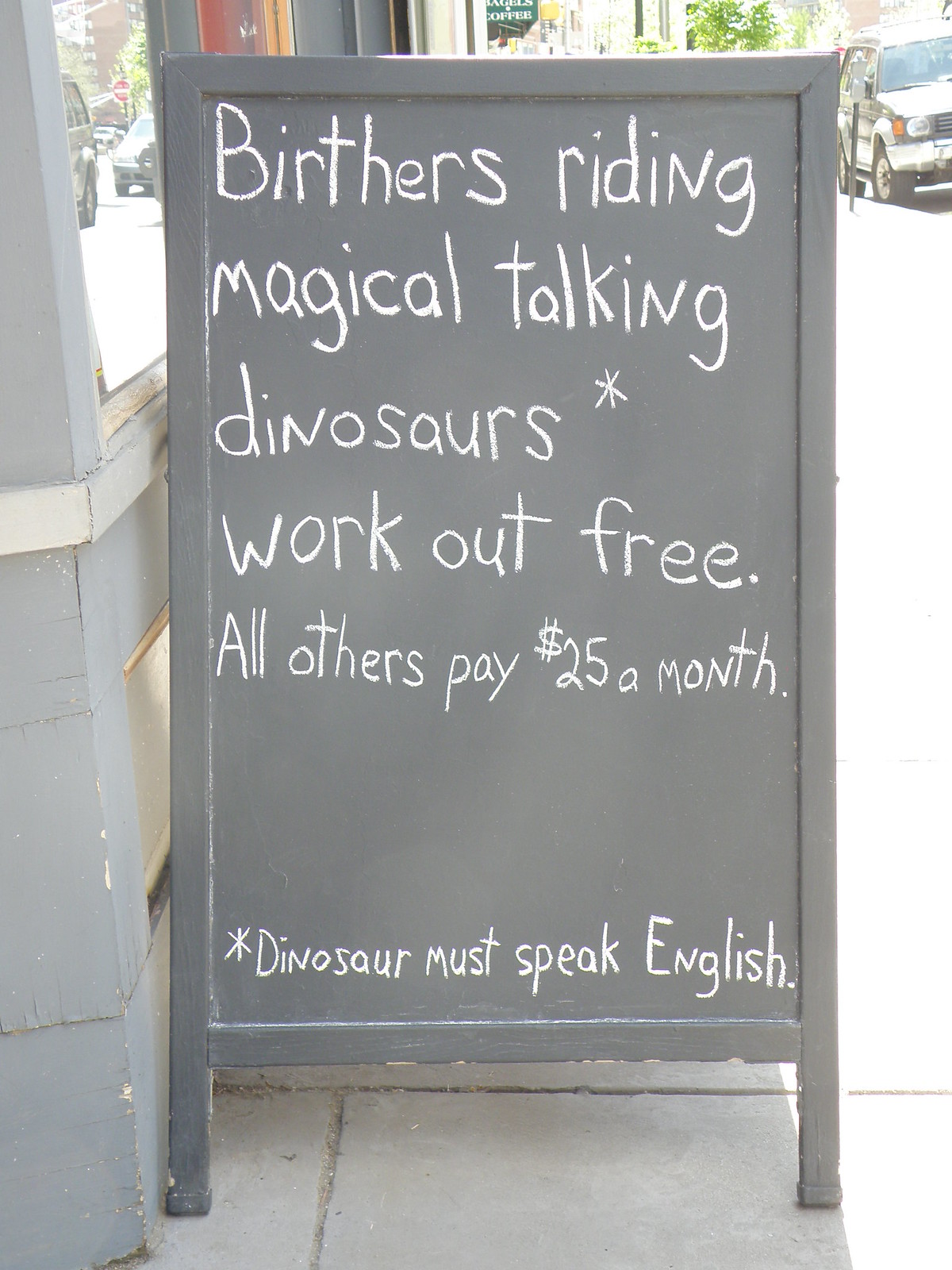The image features a chalkboard sandwich sign placed on a sidewalk with stone pavers, right next to a blue building with a visible window that offers a glimpse into the business. The black chalkboard is framed in wood and has white chalk writing that reads: "Birthers, riding magical talking dinosaurs, workout free; all others pay $25 a month." The word "dinosaurs" is marked with an asterisk, and at the very bottom, a note clarifies: "*Dinosaur must speak English." The scene is set on a bright, sunny day, and in the background, there are parking meters and several cars parked along the road, including a gray SUV and a visible car front with its headlights, tire, and wheel. There is also a sign that mentions "coffee" and a tree can be seen near the top of the image.